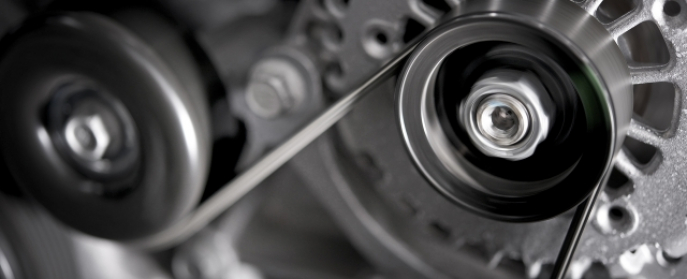The black-and-white image depicts a detailed view of a mechanical device, likely situated inside the hood of a car. The scene showcases a complex arrangement of belts and gears. On the left side, a series of belts are visible, intricately connected, and extending towards the right. Two prominent circular components, resembling gears or cogs, dominate the right side; one gear appears slightly smaller and is notable for its jagged edges and square-shaped holes near its center. This smaller gear is connected by a thin metal strip to another circular part, both apparently secured by a silver nut. The entire apparatus is bolted in place and features colors ranging from black and gray to a silverish gray, emphasizing the stark contrasts and fine details within this mechanical system.